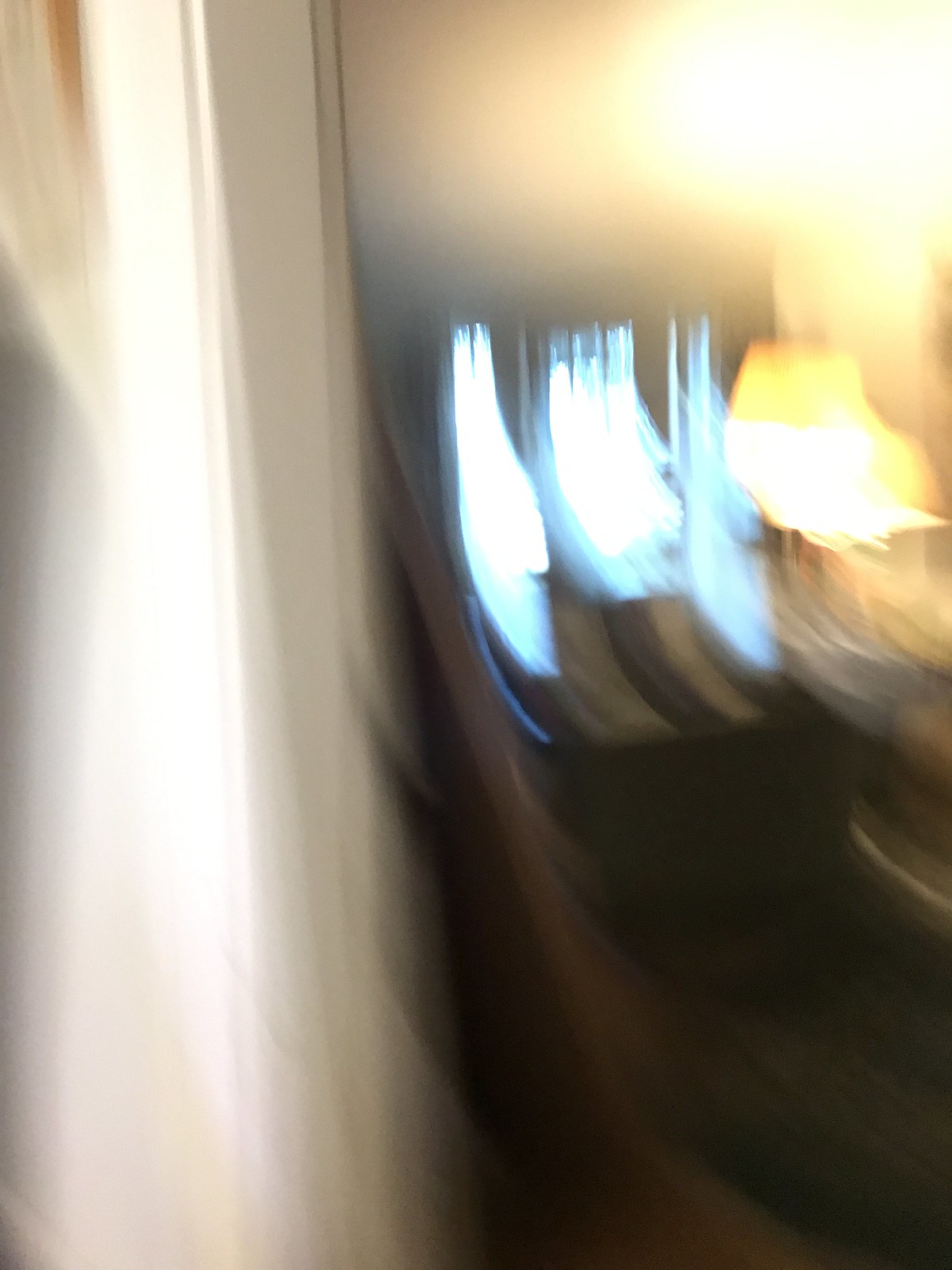This photograph is extremely blurry, suggesting it was either taken by accident or captured with significant motion. The setting appears to be the interior of a house. On the left side of the frame, there is a lamp emitting a warm yellow light. Dominating the center of the image is a door featuring three windows. The central window is shorter and positioned at the top half of the door, allowing outdoor light to filter through. Flanking this central window are two taller, narrower windows extending from floor to ceiling, also showcasing the bluish hue of the exterior light.

The left side of the image displays a white wall, adding a contrast to the overall composition. Meanwhile, the bottom right corner reveals a section of black flooring. The primary colors in the photograph include the warm yellow from the lamp, stark white from the wall, deep black from the floor, and a calming blue from the outdoor light seeping through the windows.